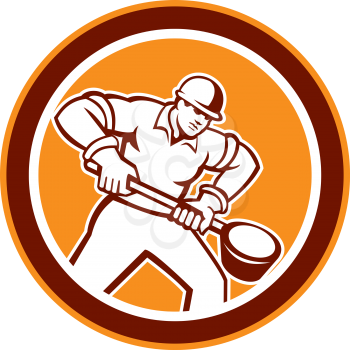The image is a round logo with a series of concentric circles: an outer circle in rust orange, a middle circle in burgundy maroon, and an inner circle in white. At the center of the logo, a muscular man is depicted in a cartoon style, wearing a white construction uniform and a hard hat. He is standing in a digging position, holding a long pole that has a bucket or barrel at the end. The man has large, muscular arms and appears to be hard at work. The overall background of the logo is a rust orange color, conveying a strong and industrious theme.